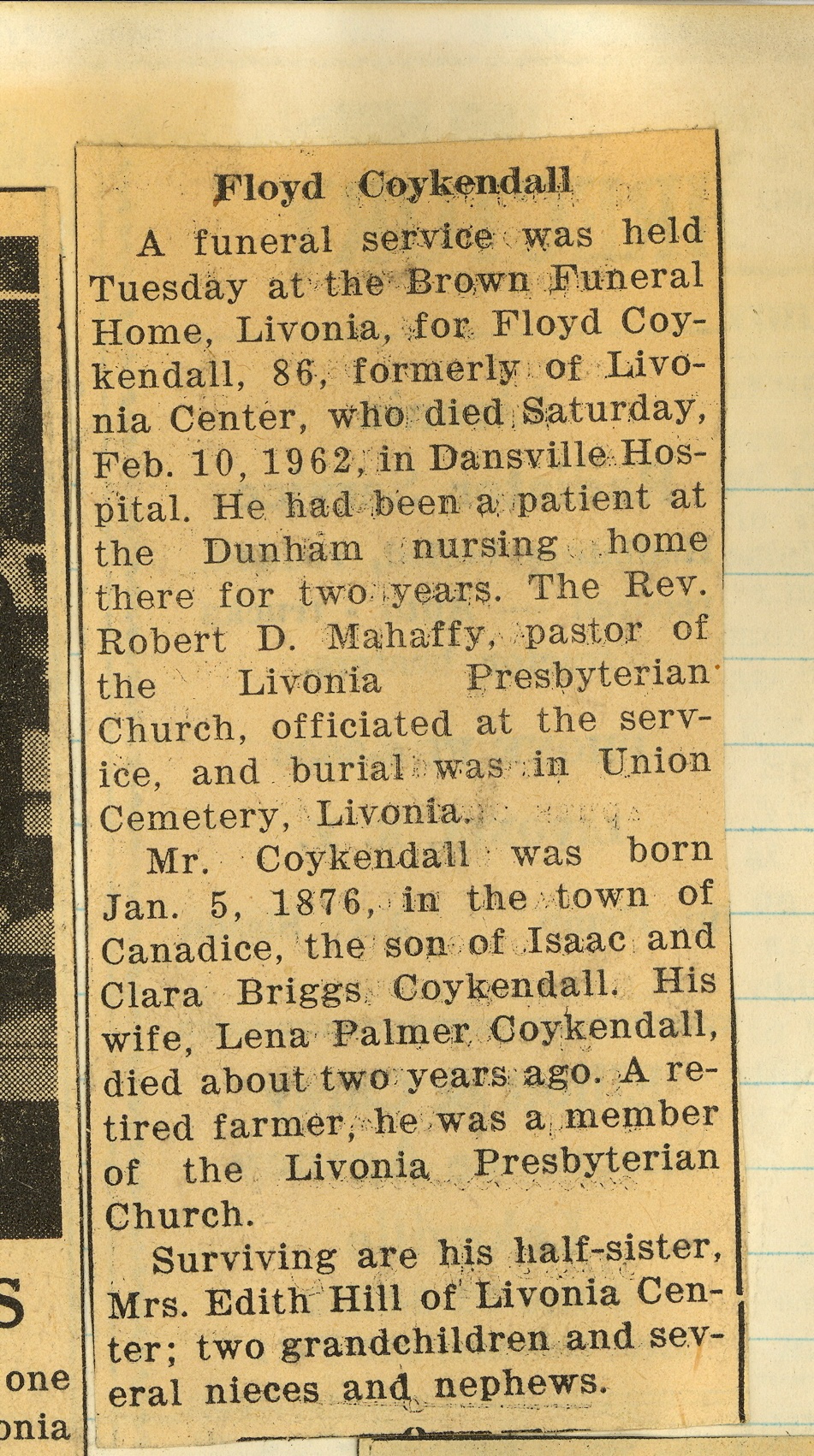This rectangular image is much taller than it is wide, featuring a clipping of an obituary from a newspaper that has yellowed and browned over time. The obituary has been pasted onto a piece of college-ruled paper, which has also aged. At the top center, in bold black print, it reads "Floyd Kuykendall," with the name spelled K-U-Y-K-E-N-D-A-L-L. The text below details that a funeral service was held on Tuesday at the Brown Funeral Home in Livonia for Floyd Kuykendall, 86, a former resident of Livonia Center, who passed away on Saturday, February 10th, 1962, at Dansville Hospital after a two-year stay at Dunham Nursing Home. The Rev. Robert D. Mahaffey, pastor of the Livonia Presbyterian Church, officiated the service, and the burial took place in Union Cemetery, Livonia. Born on January 5th, 1876, in the town of Kanedis (spelled differently as Cannadis by another account), Floyd was the son of Isaac and Clara Briggs Kuykendall. His wife, Lena Palmer Kuykendall, predeceased him by about two years. A retired farmer and a member of the Livonia Presbyterian Church, he is survived by his half-sister Mrs. Edith Hill of Livonia Center, two grandchildren, and several nieces and nephews.